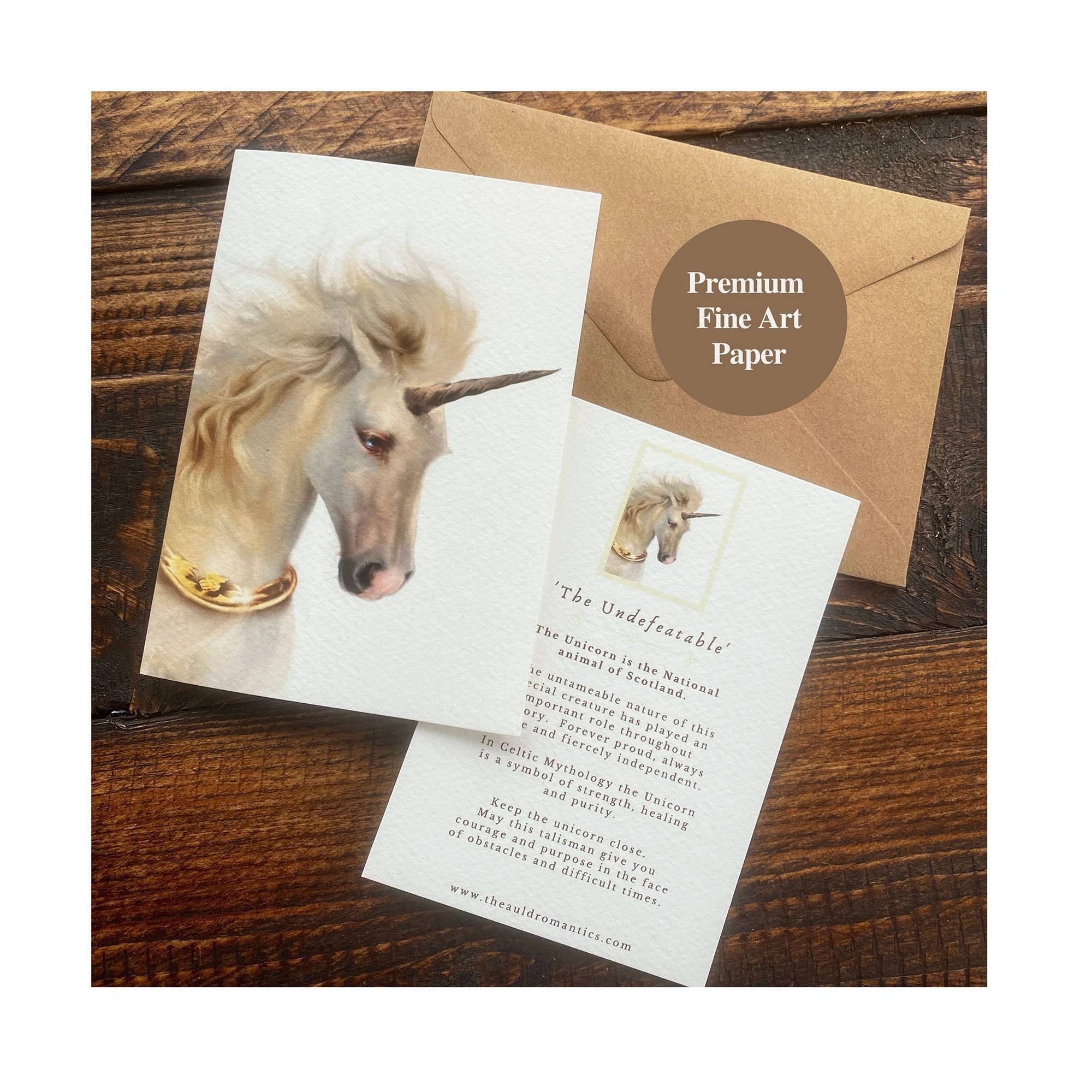This detailed photograph features a greeting card set against a dark brown wood plank background, with intricate grain and knot details. The vertical rectangular image displays two sheets of paper, angled slightly to the right. The top sheet showcases a beautifully painted unicorn on a white background, depicted from the chest up with a flowing white mane. The unicorn, adorned with a gold jeweled necklace and a prominent gray horn, faces to the right. Beneath the unicorn illustration, there's text that reads "the undefeatable," highlighting the unicorn as the national animal of Scotland. The accompanying paragraph, though partially unreadable, notes the unicorn's associations with strength, healing, and purity in Celtic mythology, encouraging the reader to keep this talisman for courage and purpose. Below this sheet is a brown envelope with a circular sticker that reads "premium fine art paper." The image is a harmonious blend of elegant art and textual details, evoking a sense of mysticism and cultural heritage.